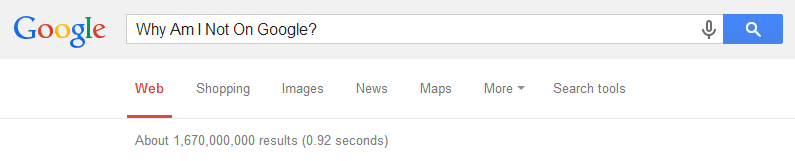This is a screenshot of a Google search results page. The user has searched for "Why Am I Not On Google," with each word capitalized. The search was performed in the 'Web' section, yielding roughly 1,670,000,000 results in 0.92 seconds. The screenshot captures Google's interface, showcasing various tabs including 'All,' 'Images,' 'Shopping,' 'News,' and 'Maps,' along with a 'More' dropdown menu and 'Search Tools.' Notably, the search results themselves are not visible in the screenshot. In the Google search bar, there's an option to use a microphone for voice search instead of typing. The blue search button with a white magnifying glass icon is also present. The rest of the page below the toolbar remains blank, indicating that only the top portion of the Google search results page is shown.